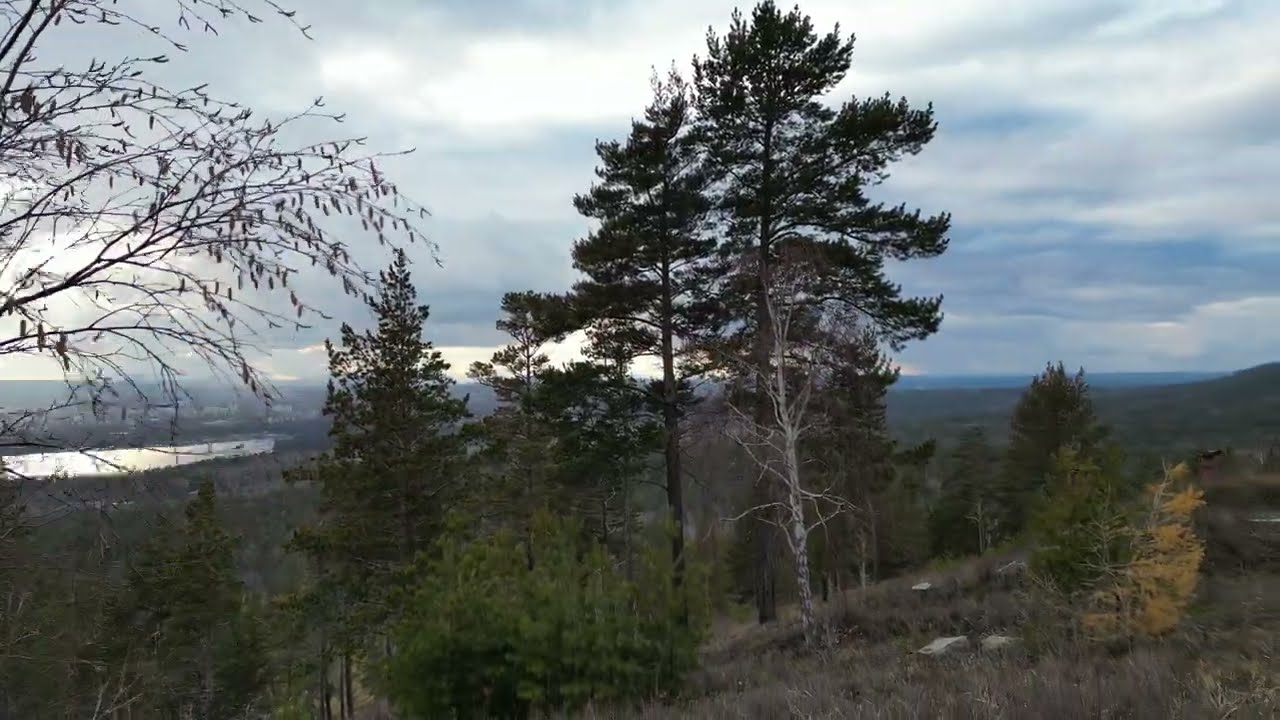The scene appears to be taken from the vantage point of a hill in the countryside, overlooking a diverse and layered landscape. In the foreground, wispy brown and green grass, along with various bushes, creates an earthy base, while leafless branches from an off-camera tree stretch into the upper left corner. Prominently featured in the middle is a tall, white birch tree, surrounded by a mix of other trees, including some pines or conifers, arranged in a line that gently slopes upward from the bottom left to the right.

Beyond the immediate trees, the land descends into a wooded area dotted with more trees, leading the eye towards a body of water—likely a lake or pond—situated towards the left side of the image. To the right, the terrain appears to remain relatively flat with gentle, rolling hills visible in the distance. The far horizon is marked by a cloudy sky, filled with layers of cirrus clouds, providing a soft backdrop to this tranquil autumnal setting.